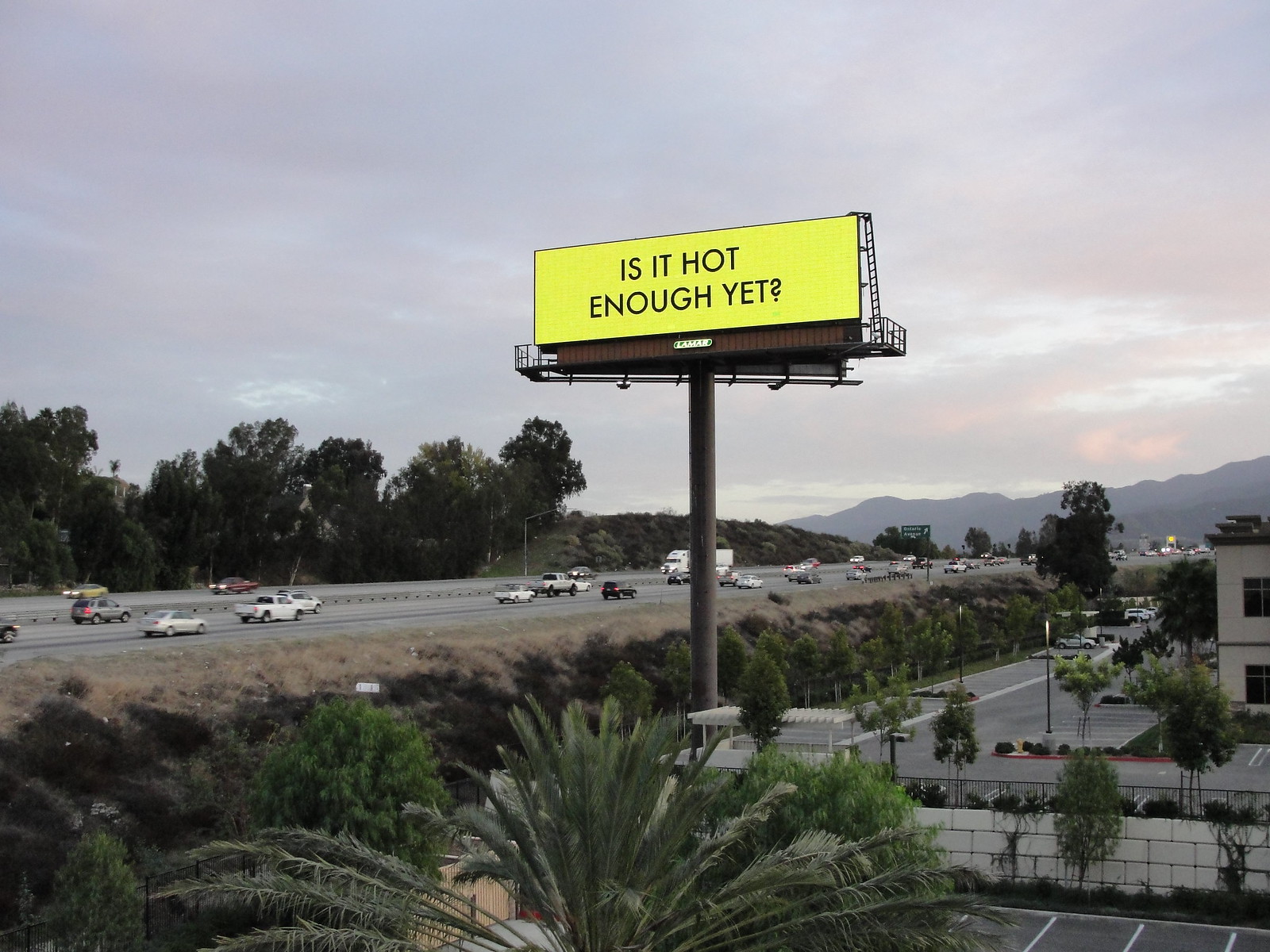This photograph appears to capture a roadside scene, likely taken from the shoulder of a highway. The foreground prominently features a busy highway with several cars in motion. In the background, a subtle, distant mountain range gracefully stretches across the horizon. To the left of the image, a dense grove of tall, vibrant green trees stands majestically. The sky is bathed in a pinkish hue, suggesting either early morning or evening light.

On the right side, a vast parking lot extends into view, adjacent to a stark, two-story white building with a flat roof. The building's minimalist, squared architecture is accentuated by its clean lines. Abutting the building is a sturdy white cinder block fence, complementing its monochromatic aesthetic. A couple of palm trees are scattered nearby, adding a touch of tropical flair to the otherwise urban setting.

In the same direction, another expansive parking lot is visible, providing further context to the urban landscape. Dominating this side of the photograph is an exceptionally tall billboard, towering at an impressive height of at least three or four stories, perhaps even taller. The billboard features a graphic with a bright yellow background and text that reads, "Is it hot enough yet?" suggesting a digitally designed advertisement.